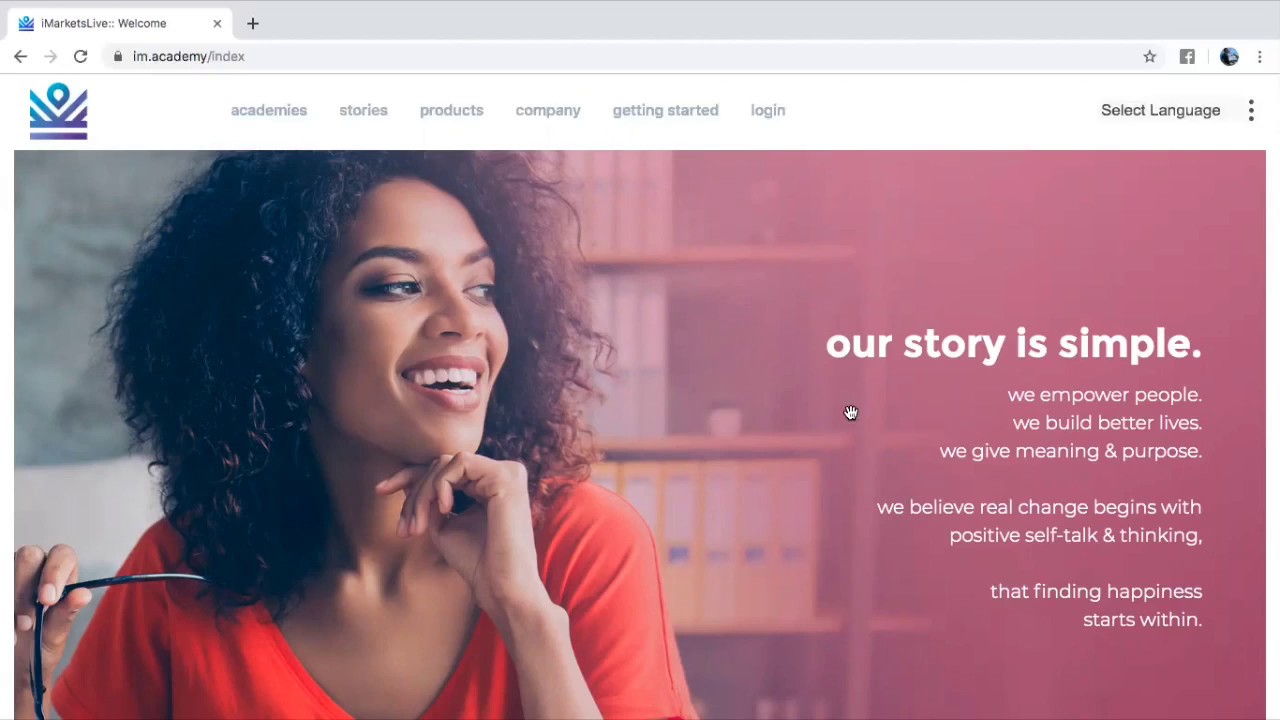This desktop screenshot likely represents a page from the Chrome browser, showcasing the im.academy.com website. The top left corner displays a gradient logo featuring blue and purple hues. At the bottom, two horizontal purple lines create the illusion of a stickman's hands and head emerging. The address bar indicates the URL as im.academy.com. The browser is currently logged in but lacks bookmarked pages, although Facebook is pinned.

On the right side of the screen, there are options including Academics, Stories, Products, Company, Getting Started, Login, and Select Language, all against a white background. The user interface also contains the Chrome menu icon with three vertical dots for additional options.

The central part of the image features an African American woman with curly hair, smiling warmly. Her left hand rests under her chin while her right hand holds a pair of glasses away from her face. Behind her are shelves, though partially obscured by a red gradient overlay.

Overlaying the image, bold white text reads: "Our story is simple." Followed by regular text that says: "we empower people. we build better lives. we give meaning and purpose. we believe real challenge begins with positive self-talk and thinking. that finding happiness starts within." These sentences are all in lowercase with periods at the end.

This website appears to belong to an academic or psychological resource organization focused on personal development and empowerment, possibly offering educational or self-improvement content designed to enhance individuals' lives and mindsets.